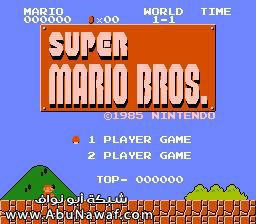The image depicts a color video game screenshot from the classic 1985 Nintendo game, Super Mario Bros. The screen is in landscape orientation and showcases the start screen of the game. Dominating the top part of the image, "Super Mario Bros." is prominently displayed in bold pink letters within a red rectangle. Below this, in white text, it indicates a selection between a one-player or two-player game, with "one player" currently highlighted. There is no score yet, with "top 000000" displayed at the very top. The player statistics show "Mario" with six zeros beneath his name and a coin counter at "0." The screen also displays "World 1-1" and "Time" without any values, indicating the very beginning of the game. 

The background features a pixelated blue sky with a green mountain on the left and a cluster of green trees on the bottom right sitting on a red brick ground. At the bottom of the screen, the URL "www.abunawaf.com" is visible, along with a line of foreign script above it. The overall style is inherently retro, emphasizing the nostalgic 8-bit design characteristic of early Nintendo games.